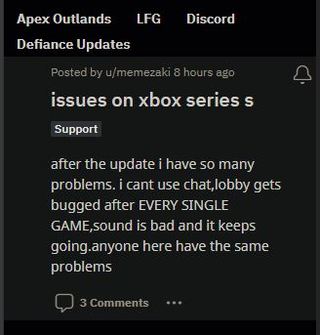The image is a screenshot from a website with a completely black background and white text. 

At the top of the image, the header displays "Apex Outlands" followed by a space, "LFG" in all capital letters, another space, and then "Discord".

Below the header, the text "Defiance Updates" is prominently displayed. Underneath this, it indicates that the post was made by "u/memezacky" eight hours ago, with a notification bell icon positioned at the far right of this line.

Directly below that information, the headline "Issues on Xbox Series S" is shown, accompanied by a lighter-colored box around the word "Support". The body of the text reads: "After the update, I have so many problems. I can't use chat. The lobby gets bugged after EVERY SINGLE GAME. Sound is bad, and it keeps going. Anyone here have the same problems?"

At the bottom, a small text chat icon with the label "3 comments" is displayed, accompanied by three horizontal dots next to it, which can be clicked to expand the comments section.